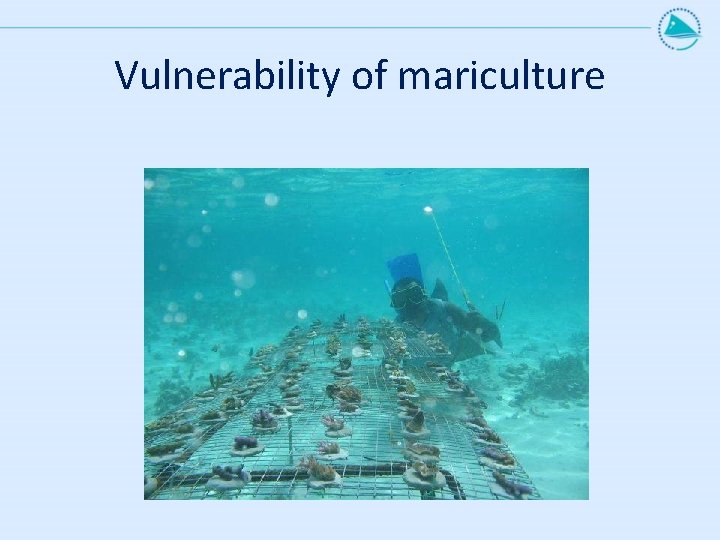The image appears to be a slide from an underwater presentation. The background is a light blue with a thin blue line running near the top, ending on the right side with a circular logo that looks like a blue triangle surrounded by small stars or waves. Directly below the line is navy blue text reading, "Vulnerability of Mariculture." The central photograph is an underwater daylight scene, featuring a man in snorkel gear examining a large wire mesh structure on the sandy seabed. The mesh system is organized with evenly spaced piping and small white circles, each hosting various types of marine life such as underwater plants, corals, or sponges. The diver appears to be conducting a scientific inspection, equipped with a long stick that has a light attached to its end.